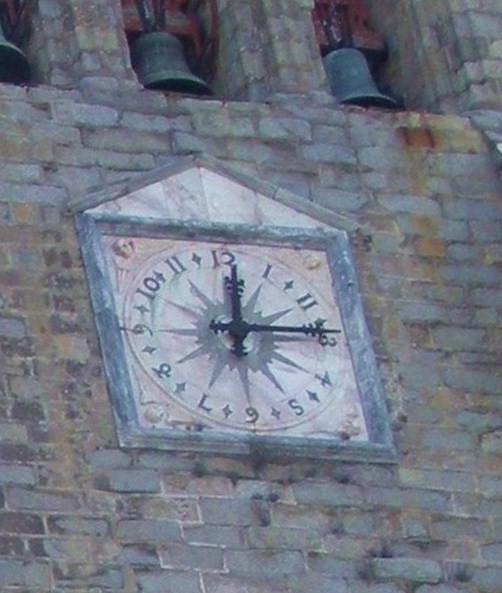This outdoor photograph captures an upward-looking view of an aged stone building, possibly a church or steeple, composed mostly of gray and tan field stones interspersed with some newer bricks. Prominently featured is a large, ornate clock set into the stone facade. Below three window arches—each housing a black, cast iron bell with the leftmost one partially cut off in the frame—the square clock is outlined in gray stone. 

Above the clock is a triangular peak also bordered in gray stone, with the triangular sections filled with a marble-like design displaying a pinkish tone. The clock's face shares this marble-ish appearance, presenting a circle in the middle with a distinctive black sunburst or star-shaped design at the center. The clock is unique with a combination of numbers; some of the numerals are Roman, specifically the I and II, while the others are standard Arabic numerals, all separated by plus signs. The time shown on the clock is 12:15. The entire structure exudes an ancient charm, enhanced by the intricate and decorative elements of the clock.